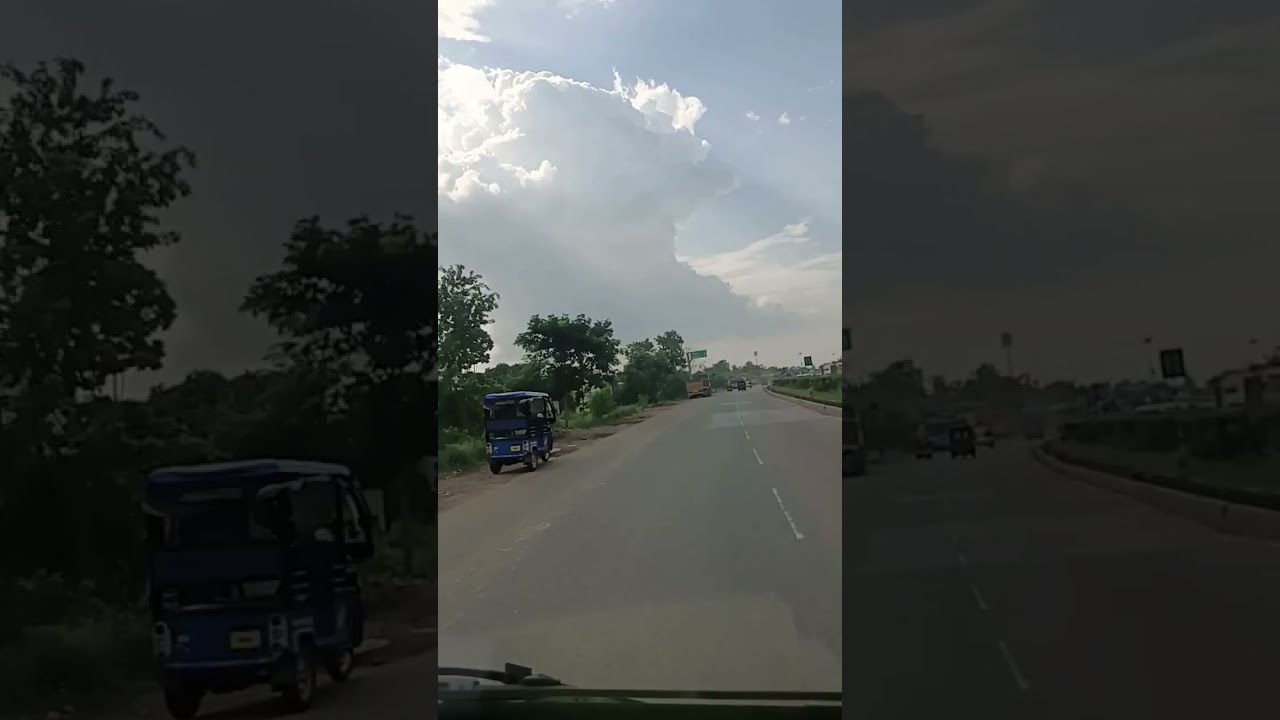In this image taken from the perspective of a vehicle on a roadway, the scene prominently features a stretch of tarred pavement with white lane markings, flanked by vibrant greenery. The middle third of the image is the clearest, where you can notice a blue vehicle, resembling a small truck or bus, parked on the right side of the road. This vehicle appears to be covered with a blue awning, offering an open-air look. On the same side, there is a close-up view of this vehicle in the left third of the image.

To the left, the roadside is adorned with tall green trees and bushes, with brown sand beneath them, adding a natural contrast to the structured roadway. The sky overhead is bright and light blue, dotted with large, white and gray clouds illuminated by the sun on the left side. On the right third, which is slightly grayed out but still discernible, there are vehicles traveling in the opposite direction and a cement barrier lined with grass. In the distance, green traffic signs and additional vehicles can be observed.

Overall, the dominant colors in the image are light blue (from the sky), green (from the foliage and signs), and the grayish-black of the pavement, creating a visually dynamic scene but devoid of specific people or animals.